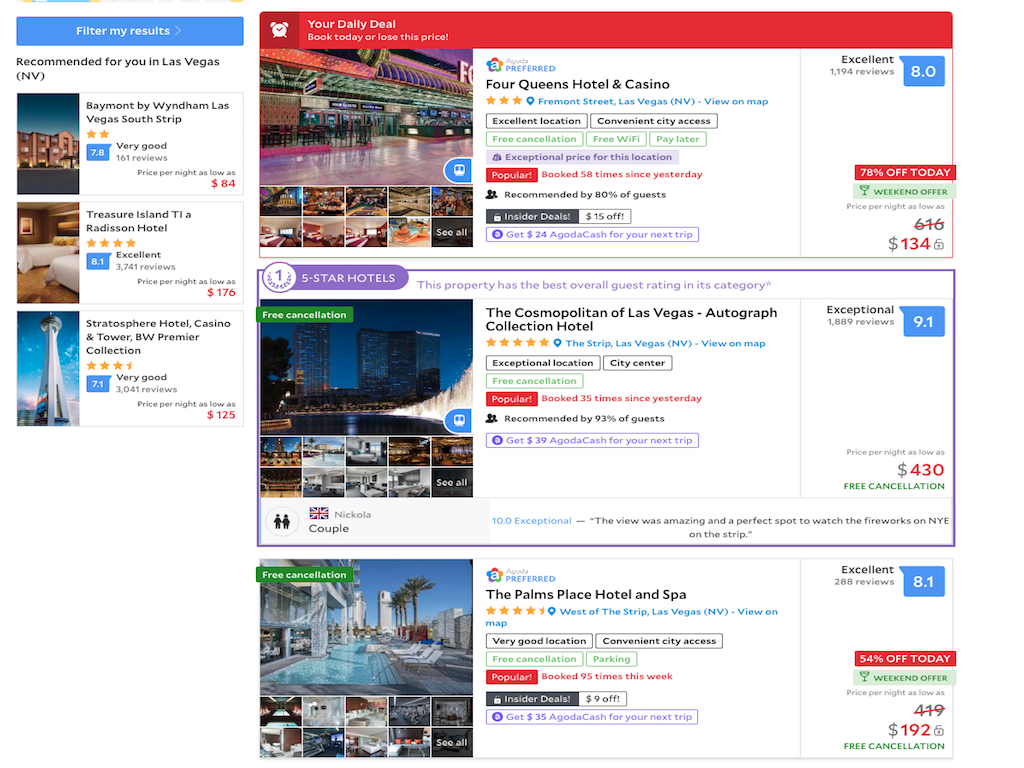The screenshot depicts a bustling desktop interface of a hotel booking website, presumably Agoda, showcasing search results for Las Vegas, NV. The left-hand column features a prominent blue "Filter My Results" button, followed by a section titled "Recommended for You in Las Vegas, NV," displaying three automatically recommended options, potentially advertisements. 

Dominating the layout, the expansive right-hand column lists three main booking options. The top option is highlighted with a striking red banner reading, "Your Daily Deal, Book Today or Lose This Price." The second listing boasts a rounded purple badge indicating, "This property has the best overall guest rating in its category," accompanied by an asterisk with undefined relevance. The final option is marked with a banner titled "Agoda Preferreds."

Each listing includes detailed information such as the name of the casino, its location with a "view on map" feature, guest ratings, and the number of reviews. Additional descriptive tags like "Excellent Location," "Convenient City Access," "Free Cancellation," "Free Wi-Fi," and "Pay Later" provide further context. Some listings also include special notes such as "Exceptional price for this location," "Booked X times since yesterday," and guest recommendations percentages. Furthermore, promotional tags like "Insider Deals, $15 off" or "Get $24 Agoda cash for your next trip" add to the informational density.

Despite the limited scope of this description, the interface is rich with user-centric details designed to aid in booking decisions.